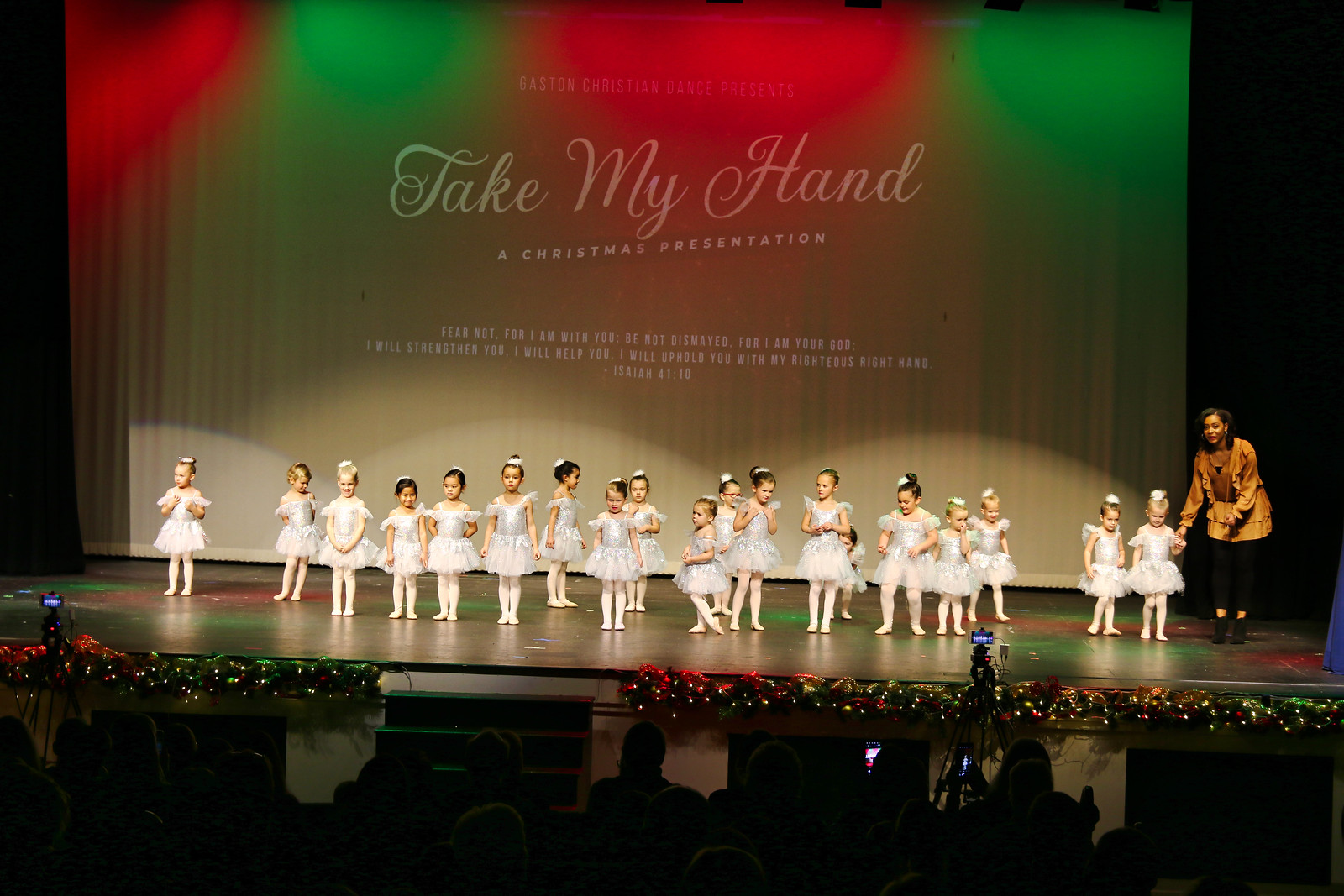On stage, about twenty little girls dressed in white or off-white ballet outfits stand in neat rows, their hair tied up in buns adorned with delicate white bows. Overhead, green and red stage lights cast vibrant hues against a tan curtain backdrop, adding a festive ambiance. The backdrop features a cursive projection that reads "Take My Hand, A Christmas Presentation," with the smaller text above saying "Easton Christian Dance." To the right side of the stage, a teacher in a gold long-sleeve top, black pants, and black shoes stands watchfully. Around the front of the stage, dimmed Christmas lights and floral arrangements add to the holiday decoration. Below the stage, a dimmed auditorium houses an audience, likely family and friends, attentively watching the performance unfold.